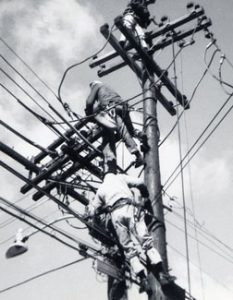This is a captivating old black and white photograph taken outdoors during the daytime using natural light. The vertical image, devoid of any specific border, is captured from a lower position, giving a dramatic perspective of the scene above. Three men, adorned in heavy-duty clothing and safety equipment, are diligently working on what appears to be telephone or utility poles, their sturdy white boots and rugged attire hinting at the demanding nature of their work.

The photograph showcases a complex web of criss-crossing wires stretching between several poles, creating an intricate and hazardous work environment. At the very top of one of these towering structures, a lone worker stands prominently, a striking silhouette against the sky filled with clouds. Below him, towards the center and bottom of the image, the other two workers are positioned on different poles, engrossed in their perilous tasks.

The background offers a muted gray sky with wisps of white clouds adding to the depth of the scene. A street lamp, distinctly visible in the lower left-hand corner, extends over the wires, further emphasizing the height and scale of the situation. The overall composition, brimming with tension and detail, beautifully captures a moment of raw human endeavor amidst the expanse of the sky.